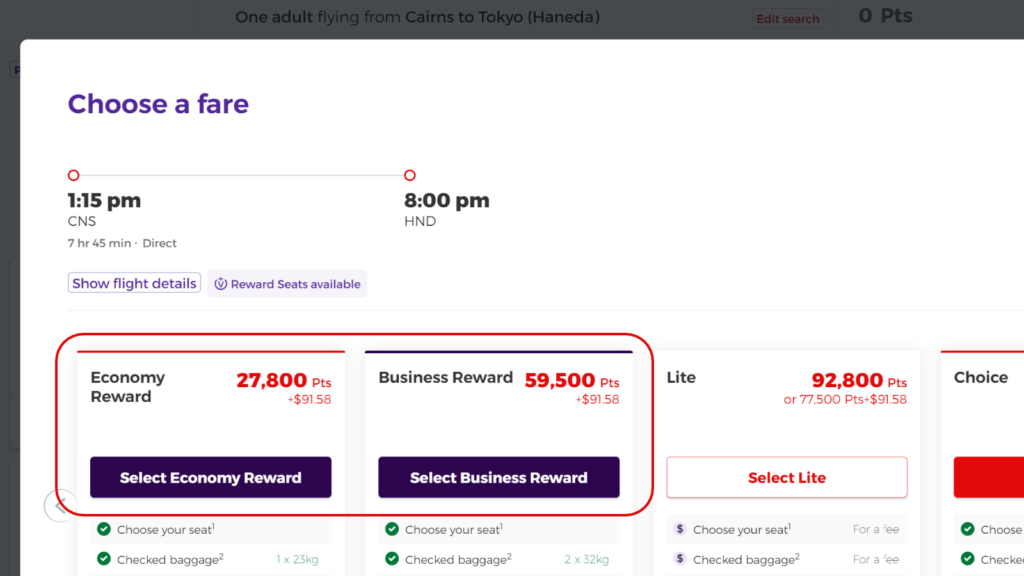The image features a user interface predominantly composed of a white rectangle on the left and upper sides, against a semi-transparent black background. The background has a grayish hue, hinting at underlying content. 

In the upper left corner of the white rectangle, the text "Choose a fare" is written in a blue-purple color. Directly below this, "1:15 p.m. CNS" is displayed, while to the right, "8 p.m. H and V 7 hours 45 minutes" is listed, indicating the duration and details of a flight.

The interface includes a white button with blue-purple text that reads "Show flight details." Below this, still in blue-purple text, "Reward seats available" is prominently shown.

Encased in a red-bordered rectangle with a white background, "Economy Reward" is offered for 27,800 points plus $91.58. This option has a blue button with white text that says "Select Economy Reward."

Next to the economy section, the "Business Rewards" option is displayed, costing 59,500 points plus $91.58. This section also contains a blue button with white text, labeled "Select Business Rewards."

On the far right, the "Lite" fare is detailed with two pricing options: 92,800 points or 77,500 points plus $91.58. This section, too, features a button that says "Select Lite."